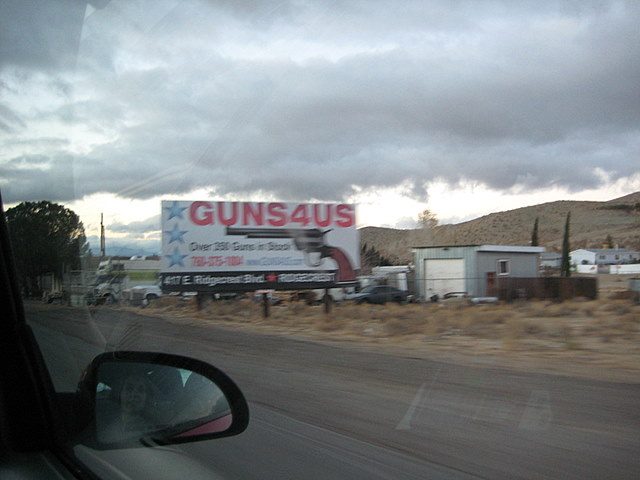The photo captures a scene viewed from the passenger side window of a car, with part of the side-view mirror and a faint reflection of the woman taking the picture visible. The sky overhead is dense with heavy, gray clouds, indicating an imminent rainstorm. The landscape suggests a dry climate, with the roadside transitioning into parched, brown grass typical of regions like Nevada. The ground is hilly and barren, further emphasizing the aridity of the locale.

The image's focal point is a prominent billboard situated near a garage. The billboard features bold, red text reading "GUNS 4 US," with "4" represented by the numeral. Below the text, there is an image of a revolver and the statement "Over 250 guns in stock." Although slightly blurry, the ad includes a phone number and a vaguely discernible address, likely 417 East Ridgemont Boulevard.

Adjacent to the billboard is a garage that appears to function as a repair center, alongside various other small buildings. Behind the billboard, a camper can be seen, further contributing to the rural and utilitarian ambiance of the scene.